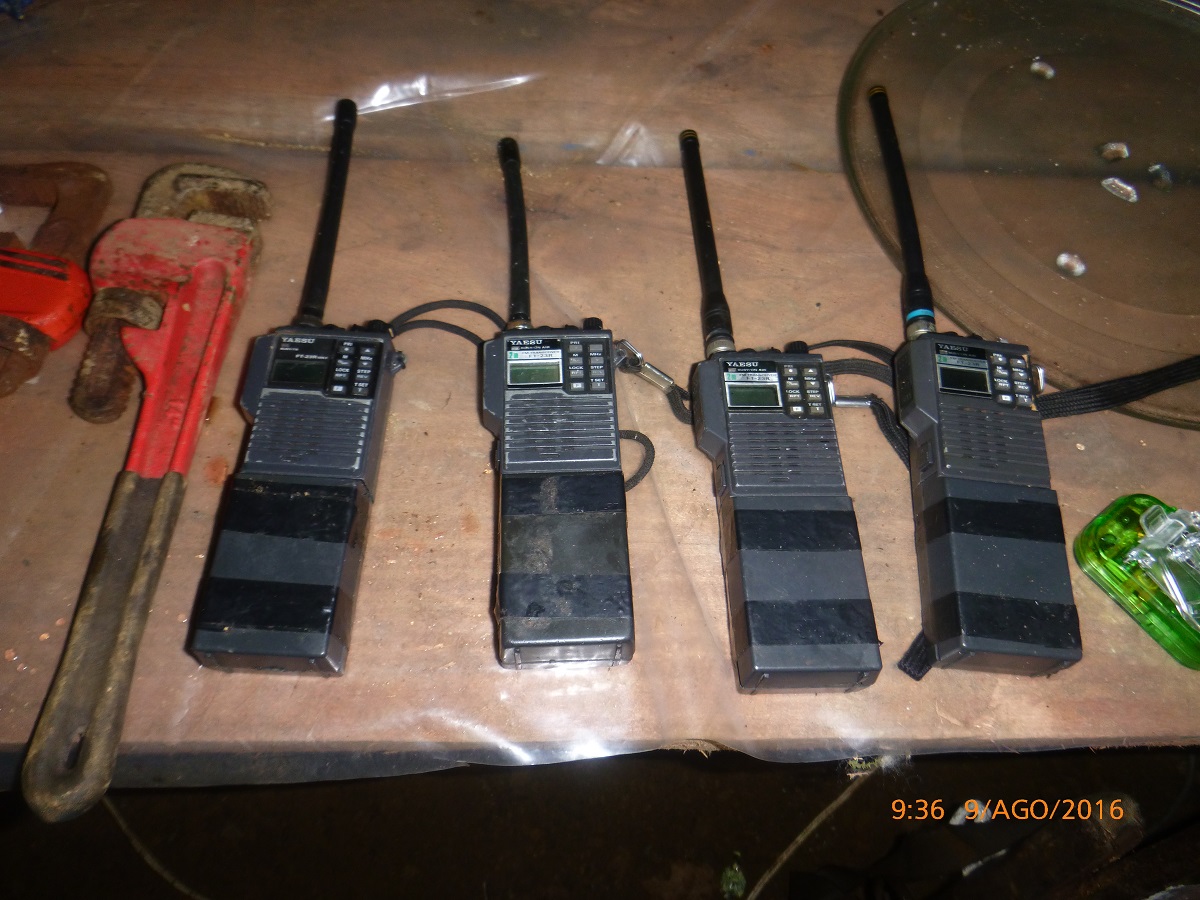This photograph showcases a set of four gray, rectangular walkie-talkies, placed on a light round table lined with a clear plastic sheet. Each walkie-talkie features a thick rubber antenna on the top left, a small green or silver-bordered display on the upper left, and several dark gray buttons on the upper right. The center of each walkie-talkie has a ridged, trapezoidal part likely functioning as the speaker grille, surrounded by two black Velcro bands. The walkie-talkies appear nearly identical, except one has a cyan blue line encircling it, possibly indicating minor differences due to lighting or wear and tear. Additionally, on the left side of the image, there are two pipe wrenches with rusted brown metal handles and red accents. In the upper right corner, a clear glass microwave tray can be seen, while in the bottom right, partly off-screen, is a bright green translucent plastic object. The photo is timestamped with orange numbers reading "9:36" and "9/AGO/2016" in the lower right corner, indicating that the date might be in a different language.